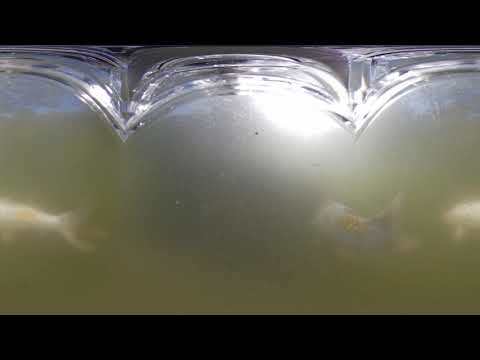This image depicts a murky fish tank with greenish-gray, almost opaque water. The tank is framed by black borders at the top and bottom, and a light shines near the beveled glass at the top, barely illuminating the interior. Despite the foggy and dirty appearance of the water, faint outlines of three fish are discernible. On the left side, the tail and part of the body of one fish are visible. Towards the right center of the image, the silhouette of a second fish can be seen. A third fish is partially captured, with only its head appearing, the rest obscured by the camera's frame. The water's coloration varies between shades of green and hints of a faded purple, making it challenging to fully discern the scene.